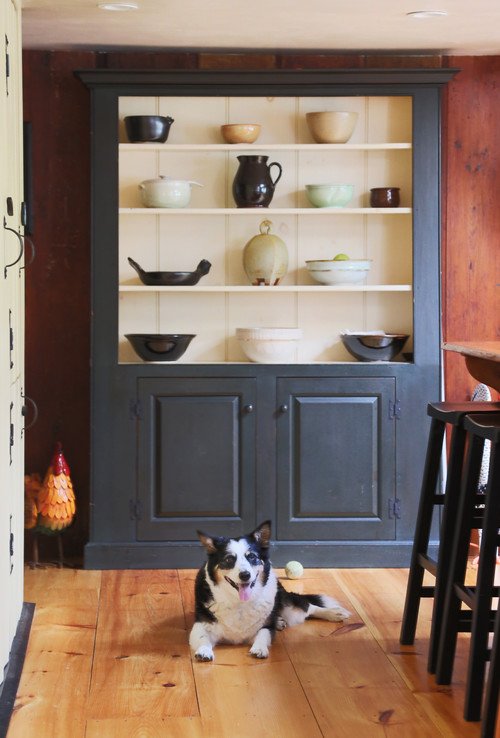Inside a cozy house, the photograph captures a charming kitchen scene. The focal point is a large, dark gray wooden cabinet with a distinct white background on its four shelves. These shelves are lined with various pottery, including beige bowls, black bowls, a black pitcher, and white bowls, creating a pleasing contrast against the white backdrop. To the left of the cabinet sits a porcelain rooster decoration. In front of the cabinet, a black and white dog with pointy ears and a white chest lies contentedly on the brown wooden floor, its tongue playfully sticking out and a small white ball just behind it. On the right side of the image are two barstools positioned next to a brown counter, adding to the rustic kitchen ambiance.